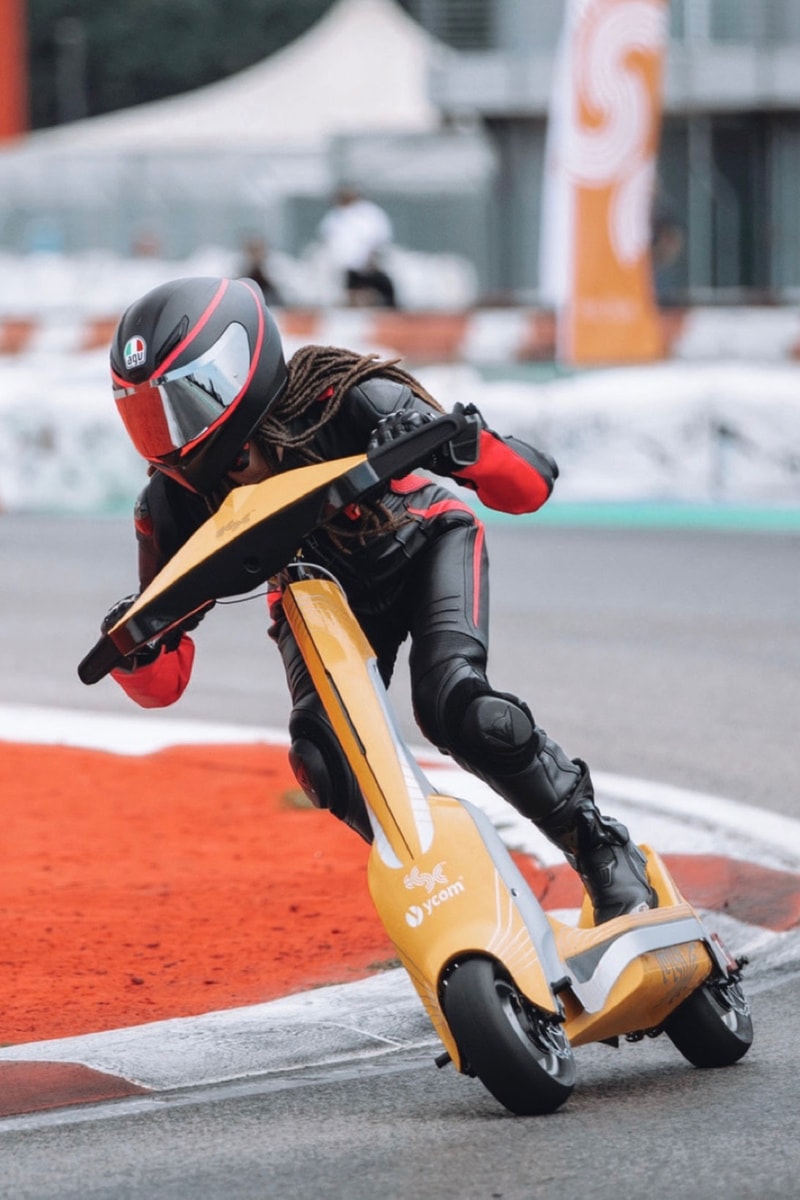The image is a detailed closeup of a racing event featuring a person on a scooter, possibly electric or motorized, captured as they round a corner on a well-paved racetrack. The person appears to be either a young girl or a man with long red dreadlocks, suggesting they are a teenager or preteen. They are equipped with a black leather riding outfit, trimmed with red accents, and are wearing a black helmet with a silver visor.

The scooter itself is a futuristic-looking, two-wheeled vehicle in shades of yellow and orange. Emblazoned on the front is a large white circle with the letters "YCLM" and an emblem resembling two mules racing each other. The rider's posture is aerodynamic, crouching and leaning forward to reduce wind resistance.

The racetrack features distinct markings, with an orange center area that is not used for racing, possibly adorned with some painted grass elements, and a green stripe around its periphery. The background is blurred to emphasize speed, heightening the focus on the racer and their dynamic motion.